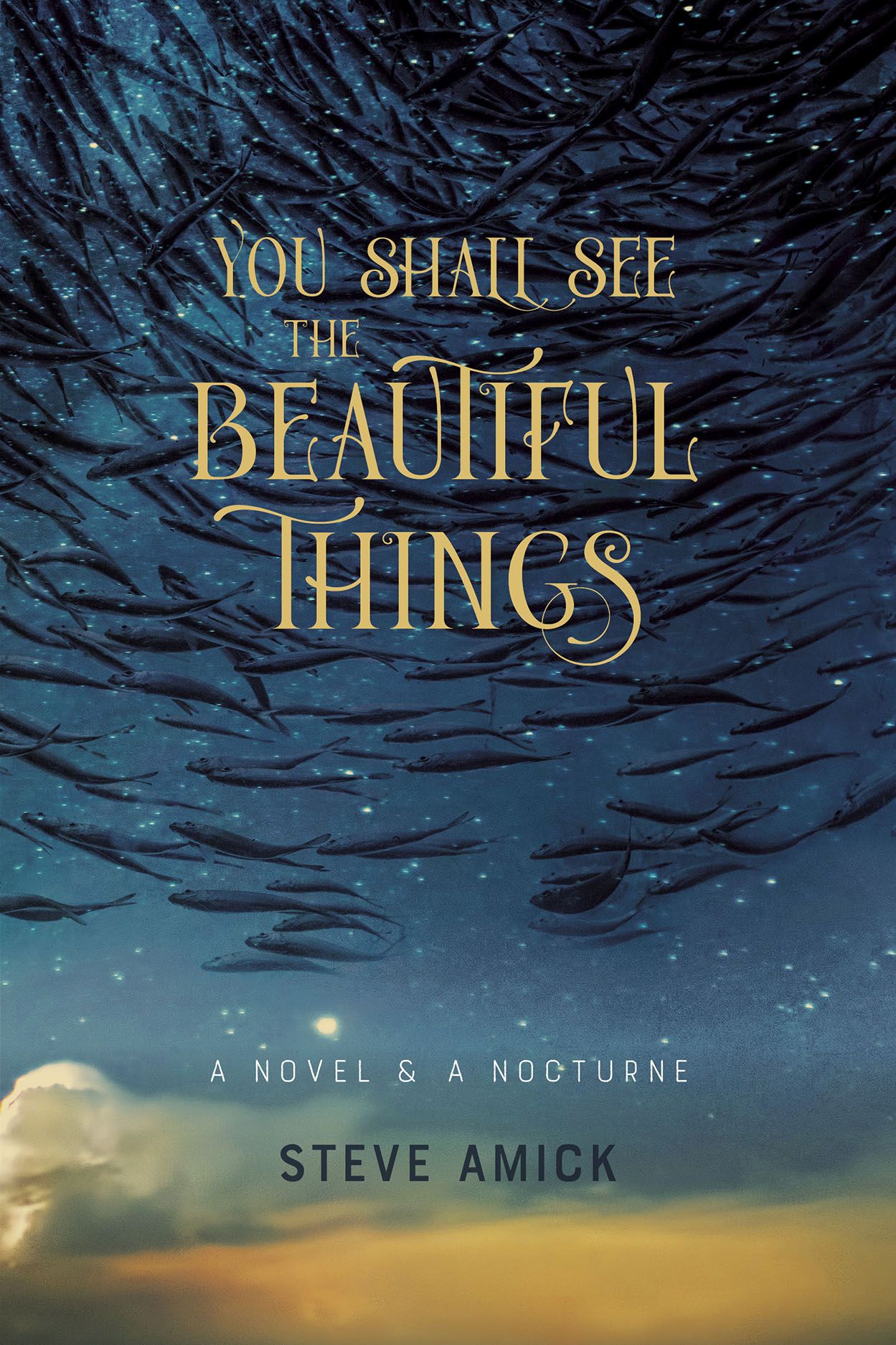The book cover of "You Shall See the Beautiful Things" by Steve Amick features a captivating blend of natural and celestial imagery. The title, rendered in an embellished beige fantasy-like font, sits prominently in the center of the cover. Below it, in smaller, white text, it states "a novel and a nocturne," with the author’s name, "Steve Amick," appearing in black. 

The background is a mesmerizing scene where a school of fish swirls through a blue ocean that progressively merges into a cloud-filled, dusk-colored sky. As your eyes move upwards, the ocean transitions into a sky with a beautiful yellowish golden hue at the bottom, blending seamlessly with white clouds. The fish, depicted in dark blue and gray shades, seem to float upwards, transitioning into what appears to be a starry night sky. The surreal arrangement creates an illusion where the fish appear to be swimming through both water and sky, juxtaposing ocean life with ethereal clouds and stars.